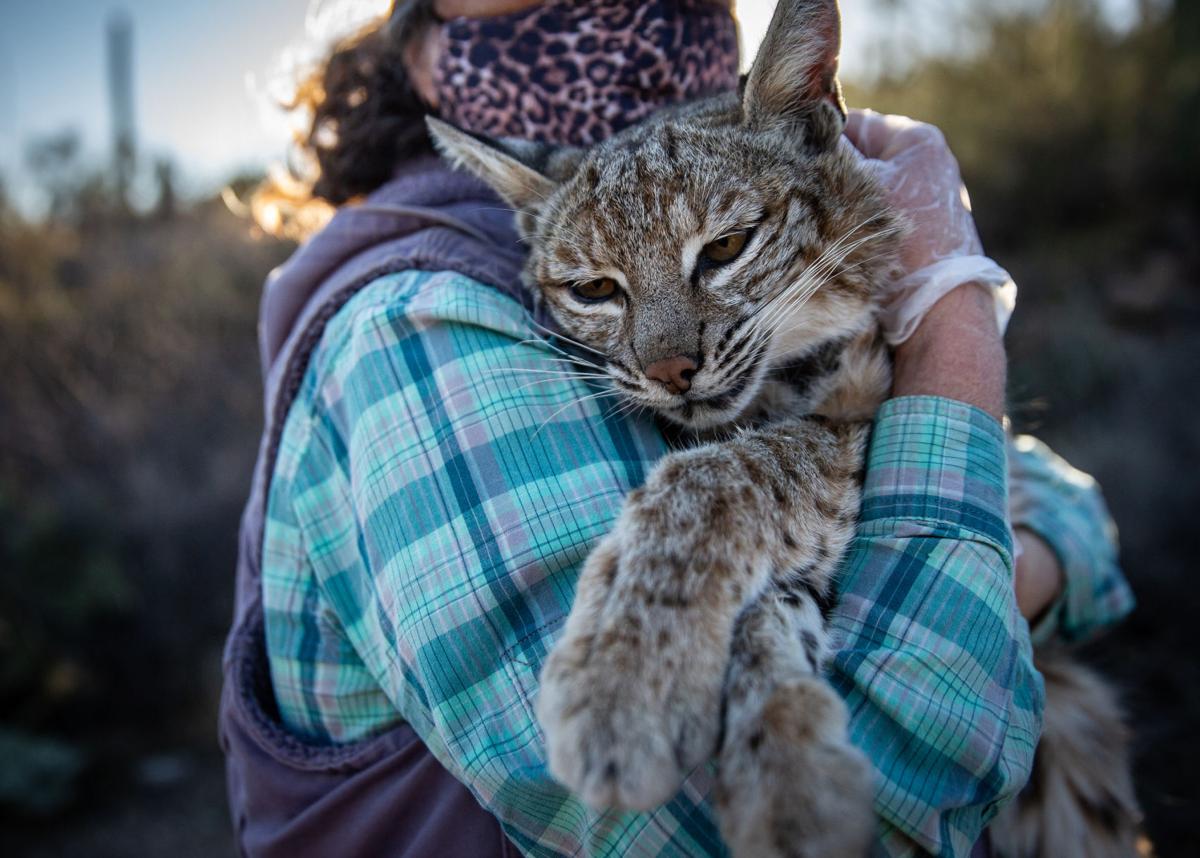In this close-up outdoor photo, a woman is prominently holding a medium-sized wild cat, noticeably larger than a typical house cat. The cat has a predominantly brownish coat and distinct, slightly larger ears, giving it a somewhat wilder appearance. The woman is wearing transparent plastic gloves and dons a distinctive face mask with a pink and black cheetah print pattern. She is dressed in a purple vest over a long-sleeve shirt, which features a plaid pattern in shades of blue, green, and purple. The blurry background reveals hints of sky and vegetation, suggesting the scene takes place outside in daylight, with the sun shining from behind the woman's head.